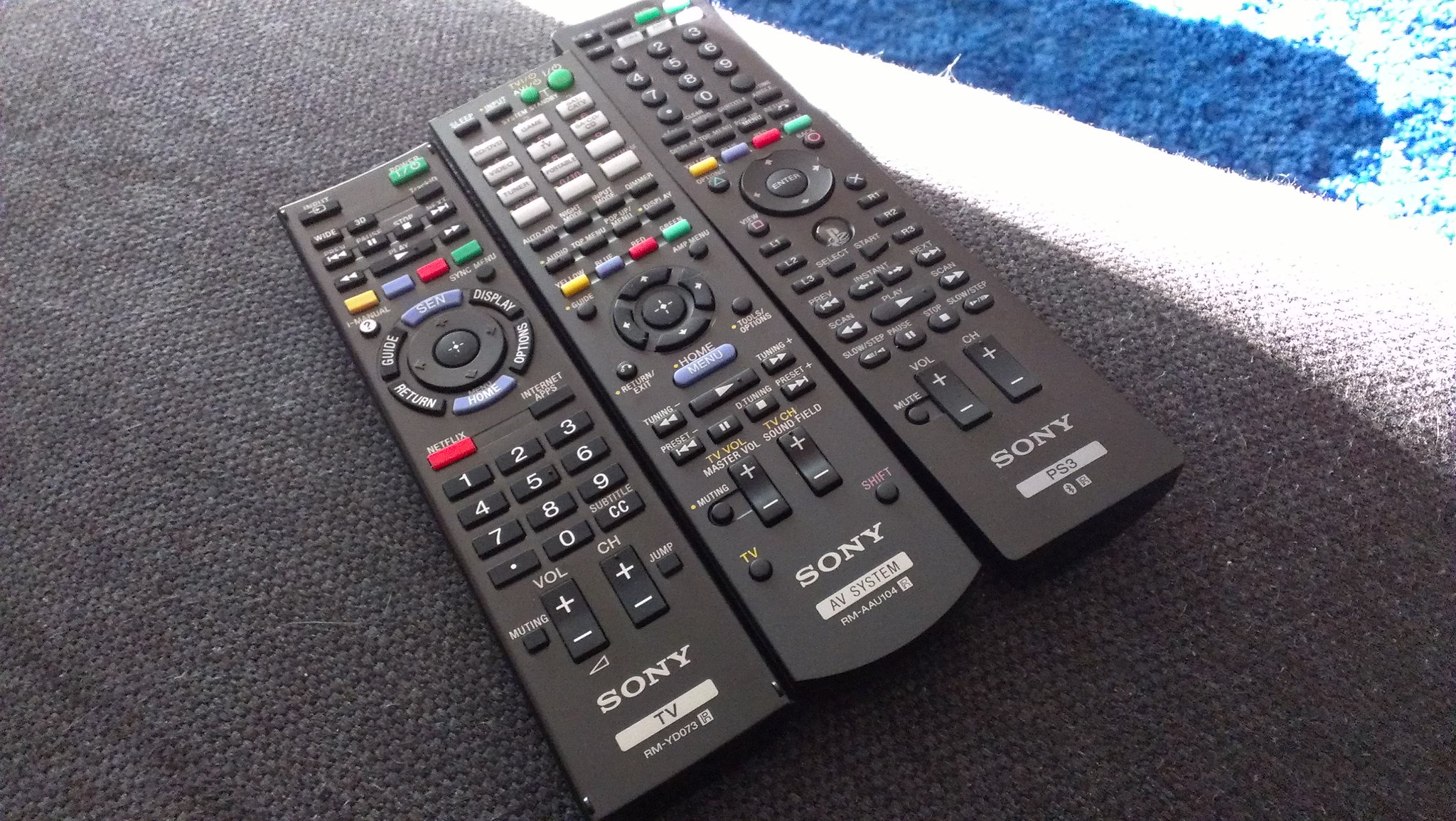This detailed color photograph features three black Sony remote controls, precisely arranged atop a gray, textured surface that could either be a couch cushion or carpet. Each remote control serves a distinct purpose: one is labeled "Sony TV," another is for the "Sony AV System," and the third is designated for the "Sony PS3." Despite their uniform black plastic construction and white printing, the remotes differ slightly in size and button layout. They are adorned with a variety of buttons, including numbers for channels, volume controls, power buttons, and other typical remote functions, with some buttons also featuring colors like yellow, blue, green, and red. The remotes rest against a distinct backdrop with a white stripe at the top and a fuzzy blue stripe. Natural light illuminates the scene from the top right corner, adding a subtle highlight to the overall composition.